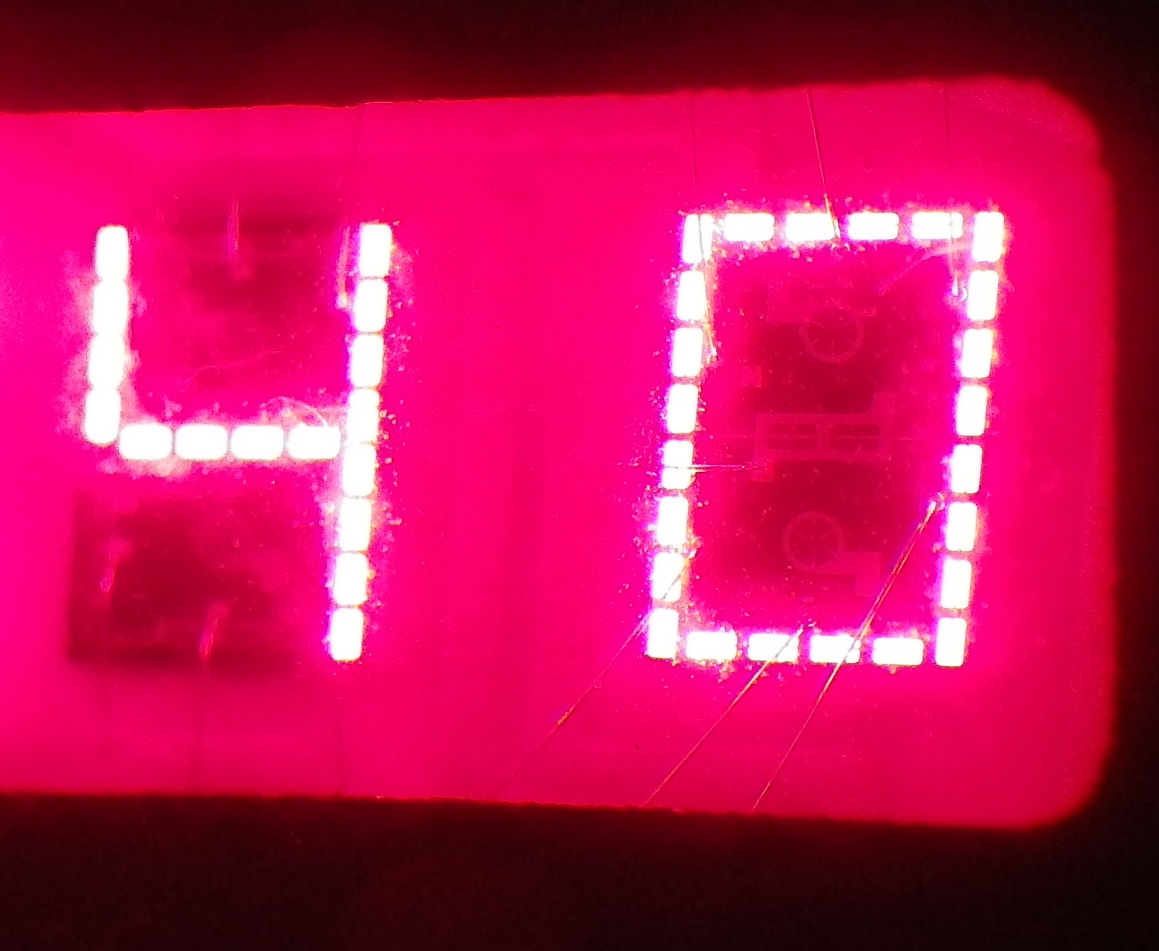This image features a digital display with a red background and white, segmented numbers composed of small rectangular dashes. The numbers on the display read "4" as the first digit and "0" as the last digit. The digital face is encased in a clear cover, revealing some of the inner workings beneath the numbers. Surrounding the display is a black frame, with the top right and bottom right corners of the digital face curving inward. The left side of the digital face extends beyond the left edge of the picture, creating a cropped appearance. The specific purpose of the display remains ambiguous, as it could belong to a clock, a dashboard, or a city sign.